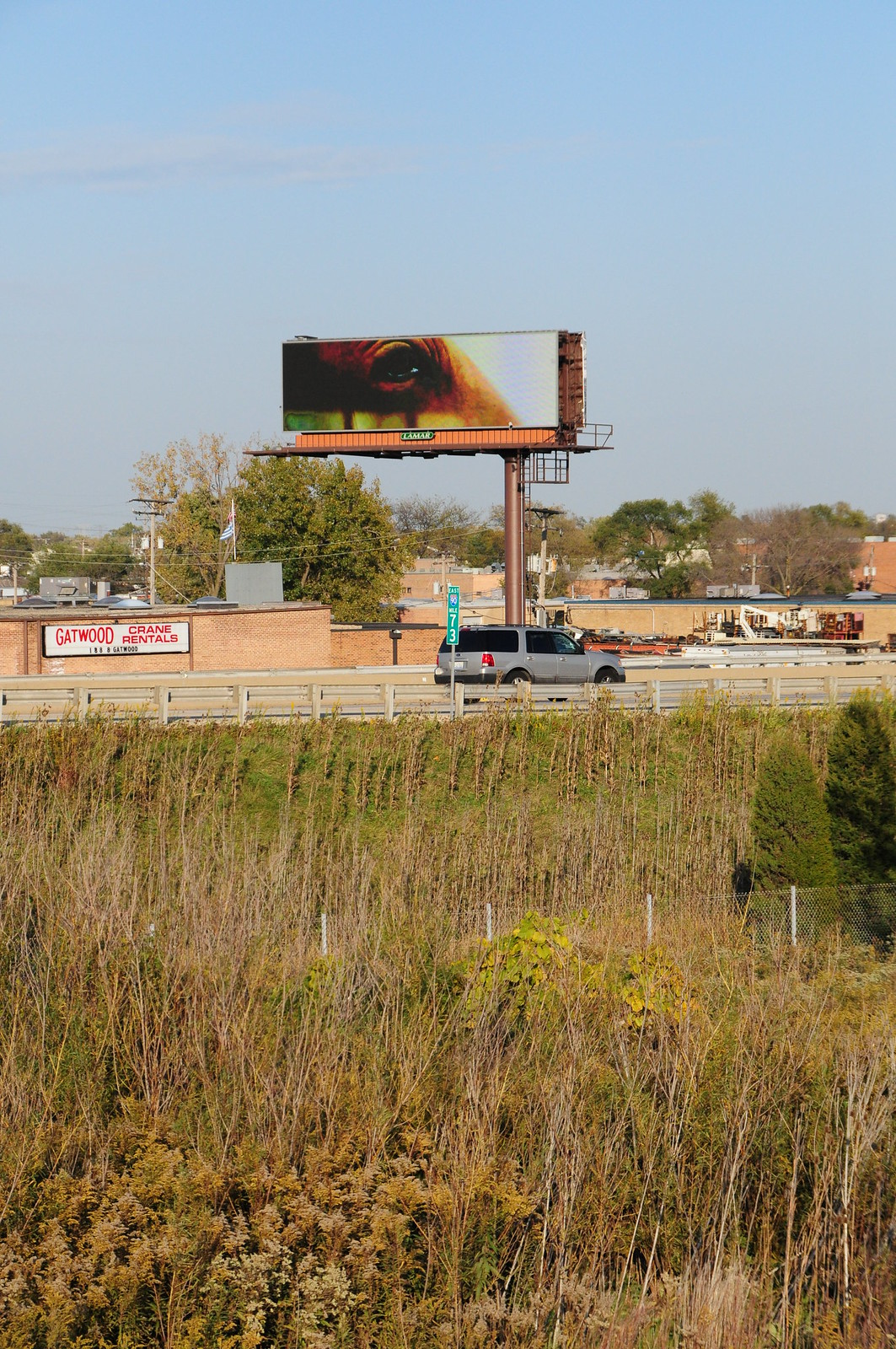In the foreground, a large expanse of dead grass, bracken, bushes, and weeds create a patchwork of browns, yellows, and greens transitioning into brown, reflecting a landscape past its prime. This rugged terrain abuts a silver roadside fence running parallel to the highway. Parked alongside the fence is a silver SUV, its metallic sheen contrasting sharply with the rustic background. 

Behind the vehicle, a building with a soft beige-peach hue stands, adorned with a white sign boasting bold red letters that read, "Gatwood Crane Rentals." The clear blue sky overhead provides a serene backdrop, subtly offset by a prominent billboard that towers above the SUV, displaying a striking image of an animal's eye. The juxtaposition of natural decay, industrial elements, and commercial signs creates a vivid tableau of a roadside setting in transition.